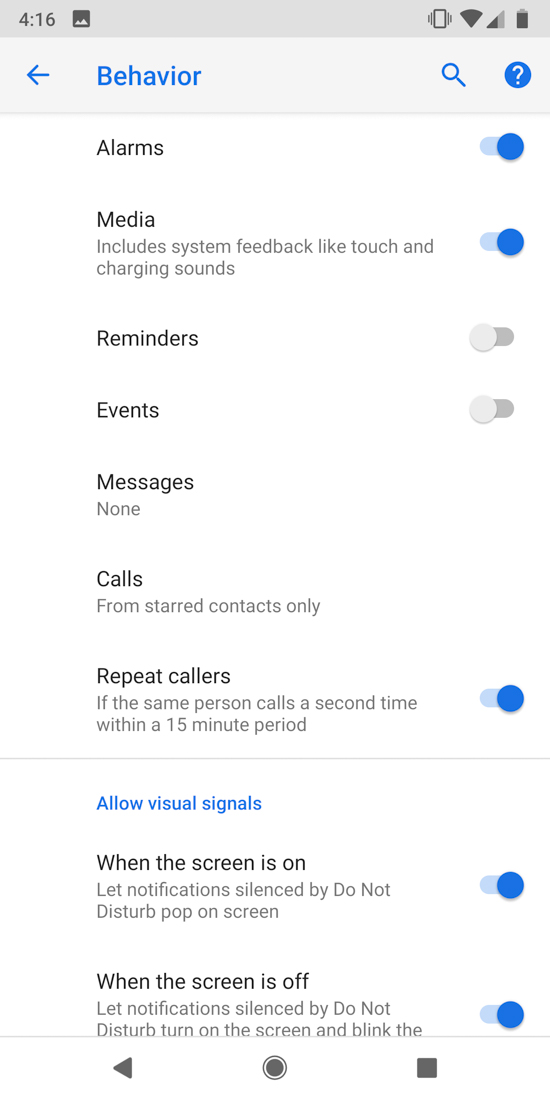The image is a detailed screenshot from a website, featuring a structured layout with various sections and indicators. At the top, there's a gray banner displaying several elements: on the left side, the number "4:16" appears next to a darker, square icon that contains a small, light-colored triangle. Adjacent to this, on the right, is a rectangular signal bar indicating cellular strength, a Wi-Fi icon, and a battery icon.

Below the banner, the background turns to a lighter gray. On the left, a blue arrow points to the left, and next to it, slightly off-center, the word "Behavior" is written in bold, blue, capitalized text. Moving further right on this lighter gray section, there's a blue magnifying glass icon followed by a blue circle with a white question mark inside of it.

The main portion of the image features a white background with various settings related to notifications and interruptions. The section titled "Alarms" is written in black text, and it lists several settings:
- Alarms: turned on
- Media: turned on
- Reminders: turned off
- Events: turned off
- Messages: none
- Calls from: starred contacts only
- Repeat callers: if the same person calls a second time within a 15-minute period, it is turned on
- Allow visual signals: appears in blue text, stating "When the screen is on: turned on" and "When the screen is off: turned on"

Each setting clearly indicates whether its corresponding feature is enabled or disabled, using a combination of text and visual cues.